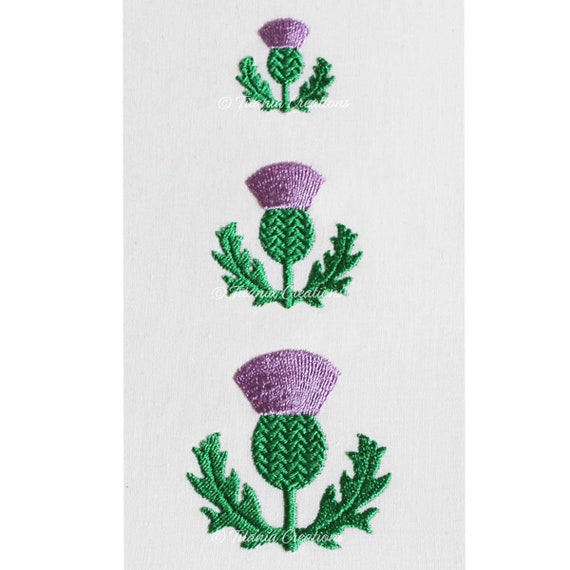In this photograph, we see a meticulously embroidered design on an off-white, vertically rectangular fabric. The embroidery, which appears to be needlepoint, features a repeated pattern of a floral motif in varying sizes. There are three identical plant-like structures aligned vertically, with the smallest at the top and progressively larger ones as you move downward. Each plant consists of a green stem with a purple-topped middle leaf, flanked by two green leaves on either side. The intricate stitching creates a detailed and textured appearance, especially pronounced in the larger designs. The background fabric is light grey or off-white, providing a subtle yet elegant contrast to the vibrant green and purple threads. Additionally, the image contains a watermark in two to three locations, indicating its proprietary nature.